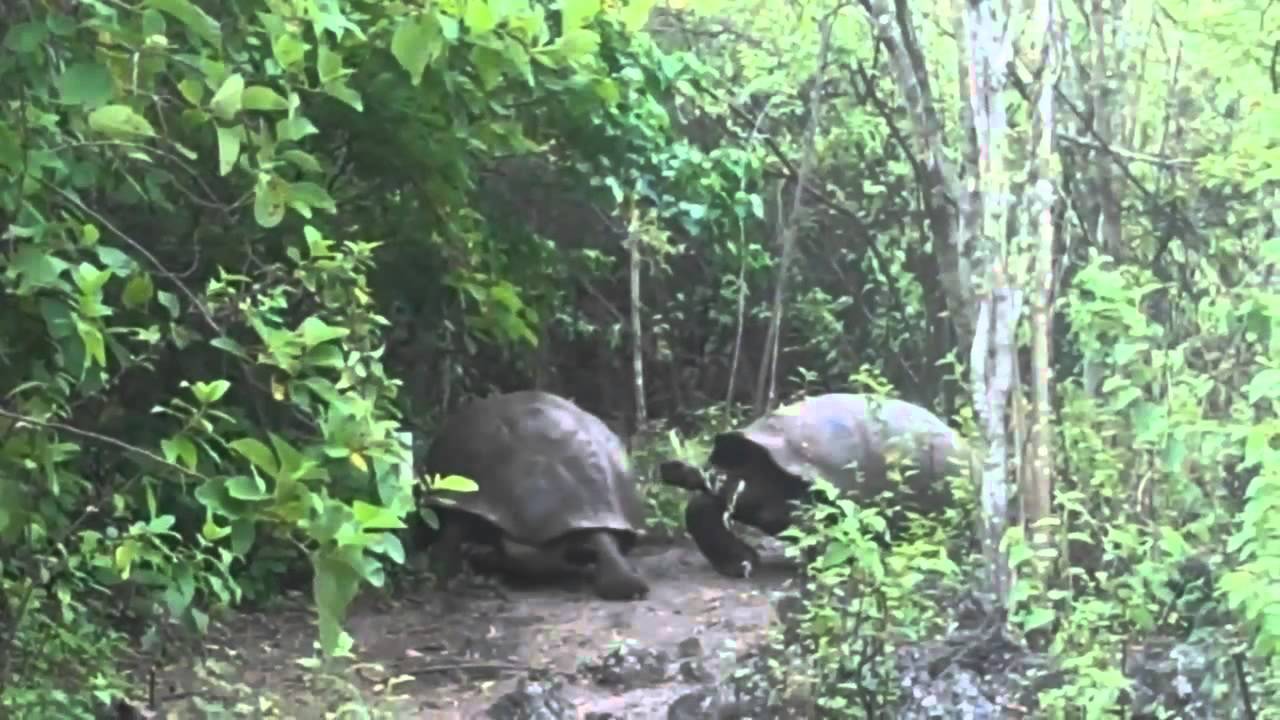This color photograph, taken outdoors in a natural setting during the day using natural light, captures a detailed nature scene featuring two large tortoises. The landscape-oriented image focuses on a back view of one dark gray or black tortoise and a side view of another, positioned close together amid a lush forest. They are not turtles; these are clearly giant tortoises with dark, weathered shells. Surrounding the tortoises are numerous hardwood trees and plants with green leaves, with sunlight filtering through the canopy, casting patches of light on the tortoises' backs. The ground beneath them appears muddy and gray, hinting at a recent rainfall that adds a wet sheen to the environment. Scattered leaves are visible on the forest floor, although the background details blur into the periphery, maintaining the tortoises as the central focal point in this vibrant outdoor scene.